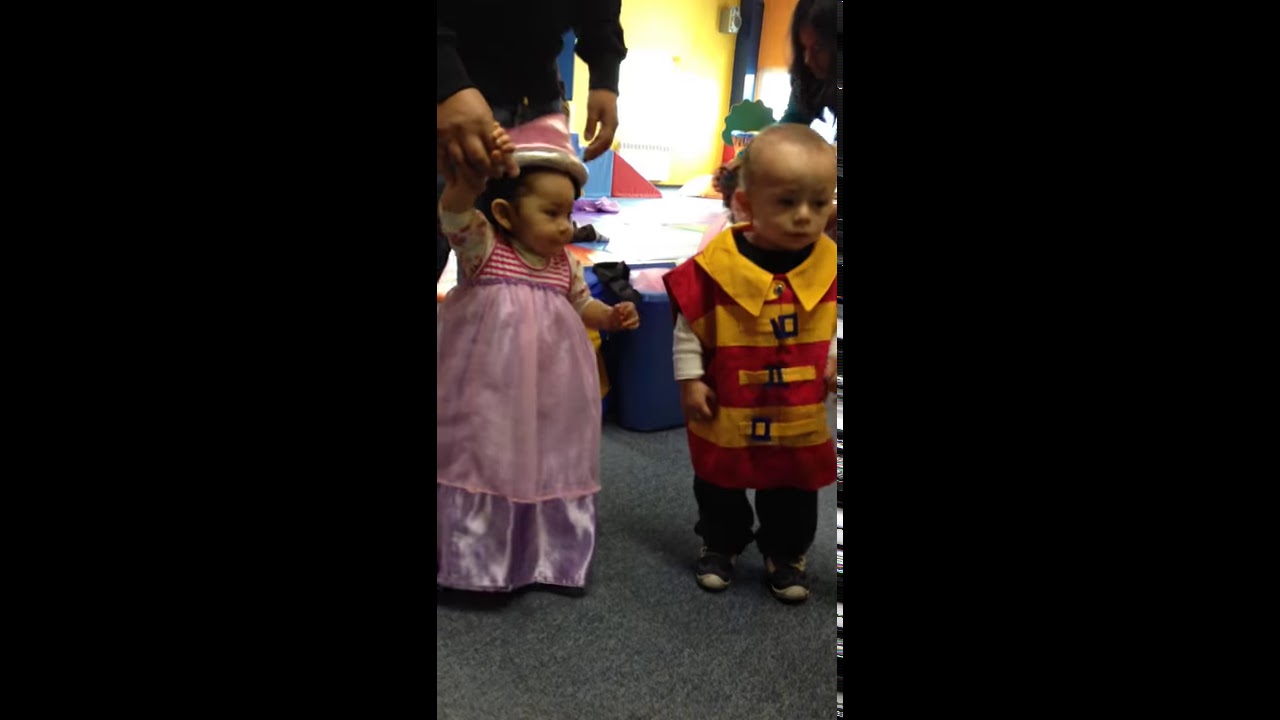A vibrant indoor scene showcases two small Asian children, a girl on the left and a boy on the right, centered on a gray-blue carpet. The little girl, dressed in a colorful ensemble of violet pants, a pinkish dress, and a red and white striped tank top, extends her right hand to an adult holding her from behind. The boy beside her wears a shirt with orange and red stripes, featuring an orange collar, and layers it over a white long-sleeve shirt, paired with dark pants and dark sneakers. The setting, illuminated with ample light, appears to be a lively child-friendly area, possibly a preschool or an amusement park, adorned with various tables, containers, and other objects in the background, where adults are seen assisting children. The colors in the scene include gray, pink, purple, red, yellow, black, blue, and green. The image is framed with darker edges, focusing attention on the lively central activity.